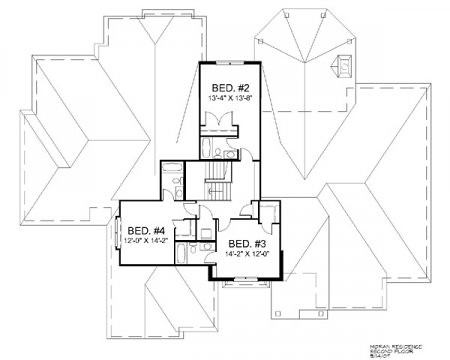This black and white image showcases a detailed architectural house plan. Central to the blueprint are various labeled rooms, precisely measured. At the top, "Bed Number Two" is delineated with dimensions of 13 feet 4 inches by 13 feet 1/4 inch. Below it, a square space likely represents a hallway. Adjacent to this is "Bed Number Three," spanning 14 feet 2 inches by 12 feet 1/4 inch. To the left, a bathroom is rendered with visible fixtures including a tub, toilet, and a door outline. To the right, another space labeled "Bed Number Four" measures 12 feet by 14 feet 1/2 inch, which connects to another bathroom at the drawing's top.

Surrounding the bedrooms, varied geometric shapes such as triangles and octagons are scattered to the left and right, possibly indicating additional structural elements or design features. At the bottom of the plan, there is some illegible writing that might provide further specifications or annotations relevant to the construction. The meticulous layout illustrates what an architect typically drafts, rendering a comprehensive overview of the house's interior spaces and their relationships.